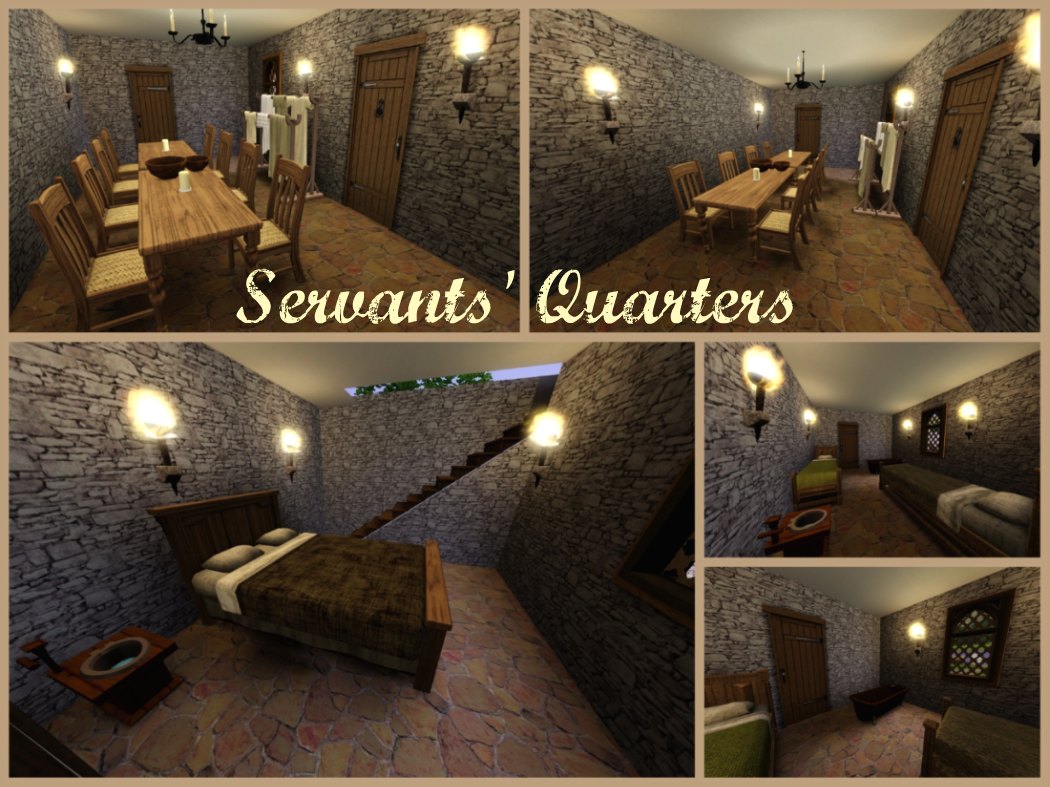This is a detailed photo grid reminiscent of a video game environment, comprised of five pictures showcasing different rooms labeled "Servants Quarters" in a script font. 

The top row features two images of the same dining hall from varying angles. The room has gray brick walls and wooden floors. The focal point is a long rectangular table adorned with two dark brown bowls and two white candles, surrounded by four light brown chairs on each side. The back wall includes a dark brown door flanked by another door and a torch on the right wall. Between the doors, a clothes rack displays garments in white, green, and brown, topped by another torch.

The larger image occupying the bottom left half reveals a gray concrete room. A brown bed with a large headboard and white pillows is positioned against the far wall, accompanied by three black-handled torches with visible flames. A wooden sink with water is placed to the left of the bed, while brown steps descend from the right side, leftward.

The right column contains two images of another room taken from different angles. Both feature gray concrete walls, a white ceiling, and four torches—two per wall. The back wall includes a window with webbing like a cage. Positioned left is a bed with a brown headboard and a bright green blanket, adjacent to a wooden door. A sink is located at the foot of the bed. Further down the right wall, a second bed with a dark green blanket and white pillow sits at the room's end. The lower image zooms in on this arrangement, with the door visible at the far end.